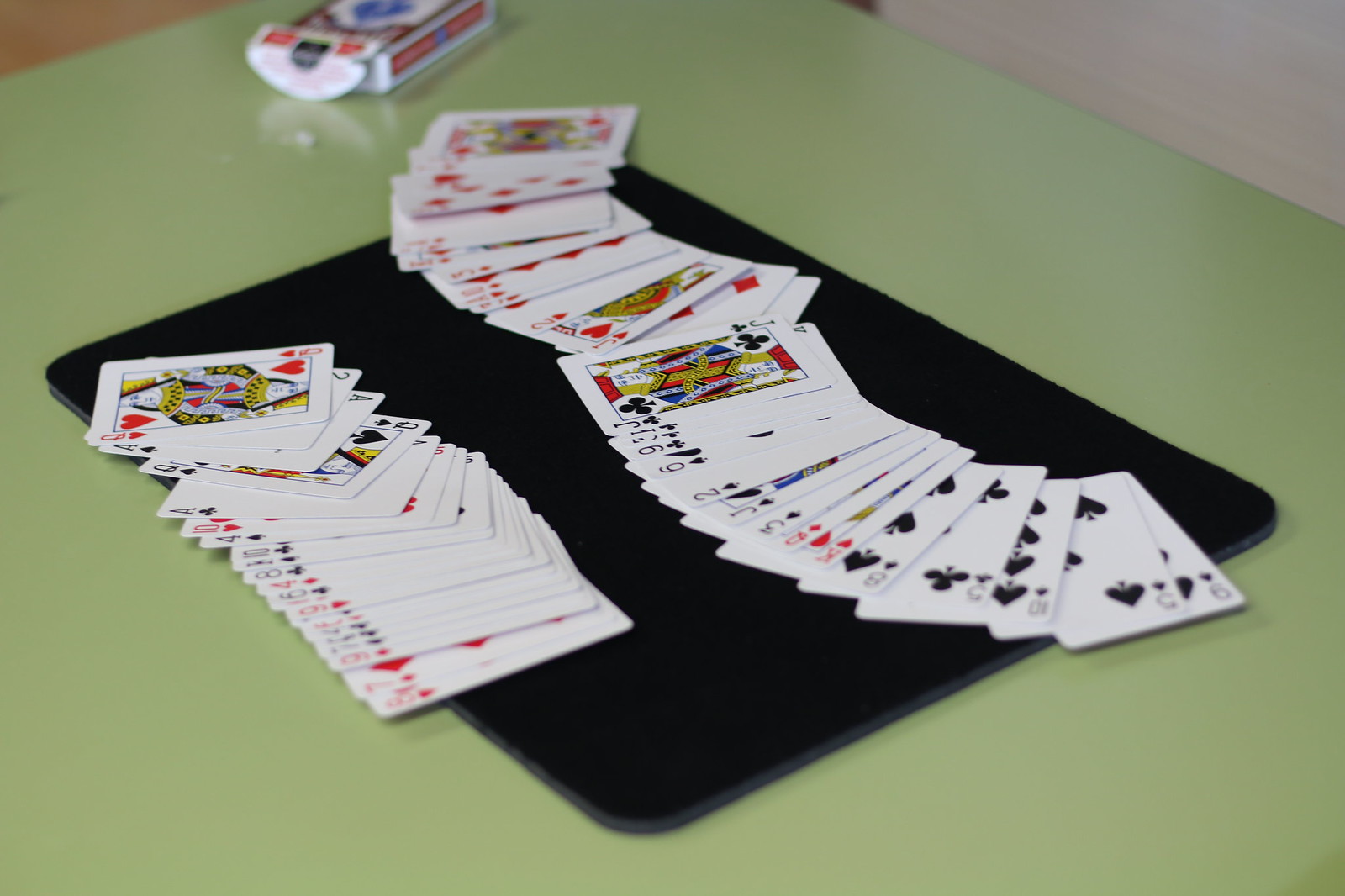The photograph showcases a light green table adorned with various playing cards. In the upper left corner of the image, a glimpse of brown is visible, while in the upper right corner, there is a touch of gray and lilac. An open playing card box lies flat at the top of the image; it is primarily white with red and blue accents. A black mat, reminiscent of a thick, cushiony mouse pad, is placed diagonally on the table, serving as the primary surface for the cards.

The mat is filled with a scattering of playing cards, which are spread out in a detailed, methodical fashion. Starting from the left-hand side at what appears to be the top of the mat (despite it being the bottom in position), approximately a third of the cards are evenly dispersed, though a few near the upper edge appear slightly disheveled. As the viewer's gaze moves downward (visually upward due to the diagonal mat position), the remaining cards form a gentle arc, maintaining an organized spread. Notably, when examining about two-thirds of the way through the spread, a distinct arc of red cards appears, suggesting a deliberate sorting method. These red cards are also meticulously splayed out, adding a touch of intrigue to the arrangement.